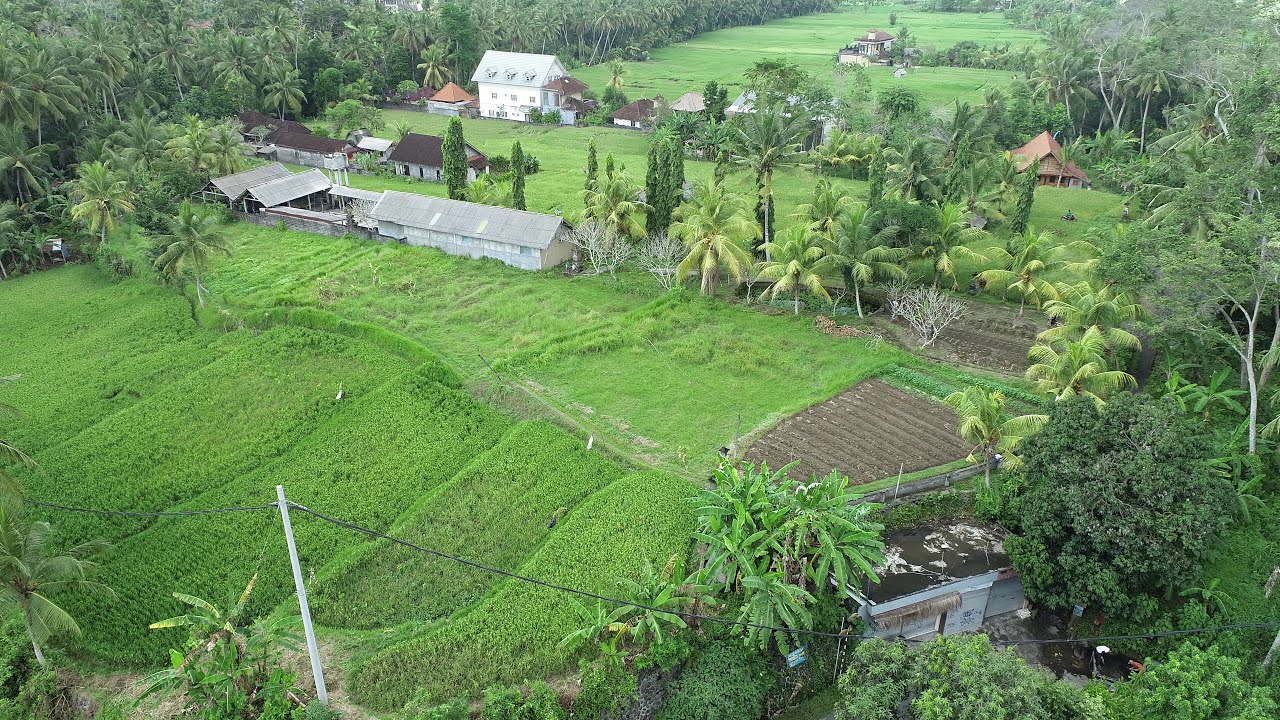This is an aerial photograph taken by a drone, showcasing a lush, tropical farming area that appears to be situated in an Asian country such as Vietnam, Laos, or Thailand. The vibrant green landscape is dominated by dense palm forests surrounding expansive rice paddies in the foreground. The rice paddies are meticulously arranged and bordered by an abundance of palm trees which characterize the tropical climate, indicating the region receives ample rainfall. At the center of the image, there are several well-maintained farm buildings, including a prominent white, two-story farmhouse with an A-frame roof and three small windows protruding from the roofside. Nearby, another house and a cultivated garden area, prepared for planting, can be seen. Additional buildings, potentially a greenhouse or barn, are visible in the distance. The flat, green patches of farmland lie amidst the thriving jungle and various tropical trees, reflecting a harmonious blend of natural and cultivated land. Electrical poles suggest that the area, although predominantly natural, is not entirely remote. The overall scene captures the vitality and productivity of a farming community thriving in a verdant, tropical environment.